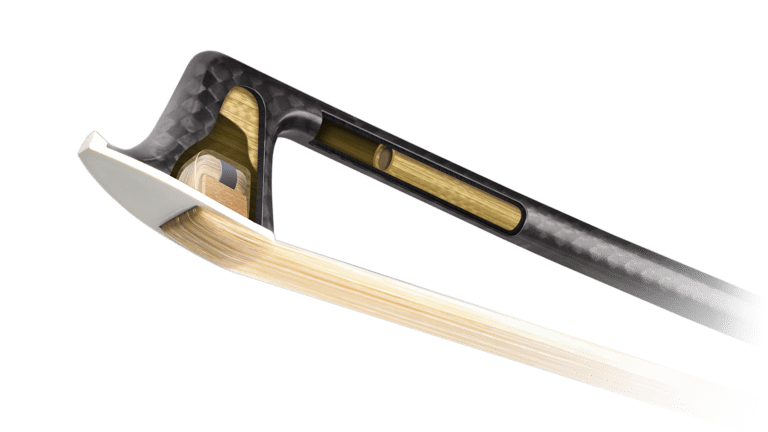This close-up photograph showcases a peculiar object with various recognizable features, though its exact purpose remains ambiguous. Dominating the image is a long black pole-like stem, which has a cutaway section revealing an internal bamboo or wooden tube. Attached to this stem, there's a long wooden handle, extending from a section that includes a pointed metal bit resembling the underside of an iron. The metal part gives the impression of a ski with cutaway sections. Despite initial impressions suggesting it could be a hand saw, a violin bow, or even an axe, the object's true identity is unclear.